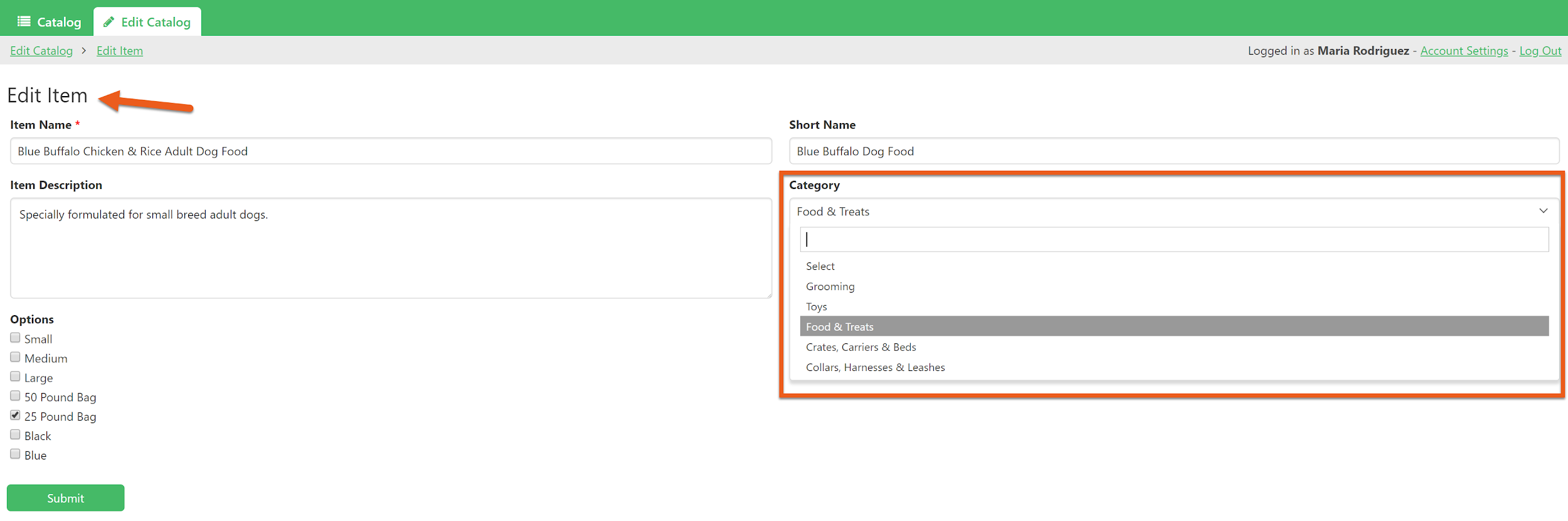The image is a detailed screenshot from a dog food company's website, showcasing a catalog editing interface where the logged-in user, Maria Rodriguez, can modify items. The interface prominently features a red arrow pointing to an "Edit Item" button. The editing options include fields for item name, item description, options, short name, and category. The category section is highlighted with a red-outlined square and lists several options, including Select, Grooming, Toys, Food and Treats, Crates, Carriers and Beds, and Collars, Harnesses, and Leashes. Below the editable fields, there's a green "Submit" button, visually matching the green background of the catalog title at the top of the screen. Additionally, at the top-right corner, it shows that Maria Rodriguez is logged in, with options for account settings and logout. The clean and organized layout is set against a white background, ensuring ease of navigation and clarity.